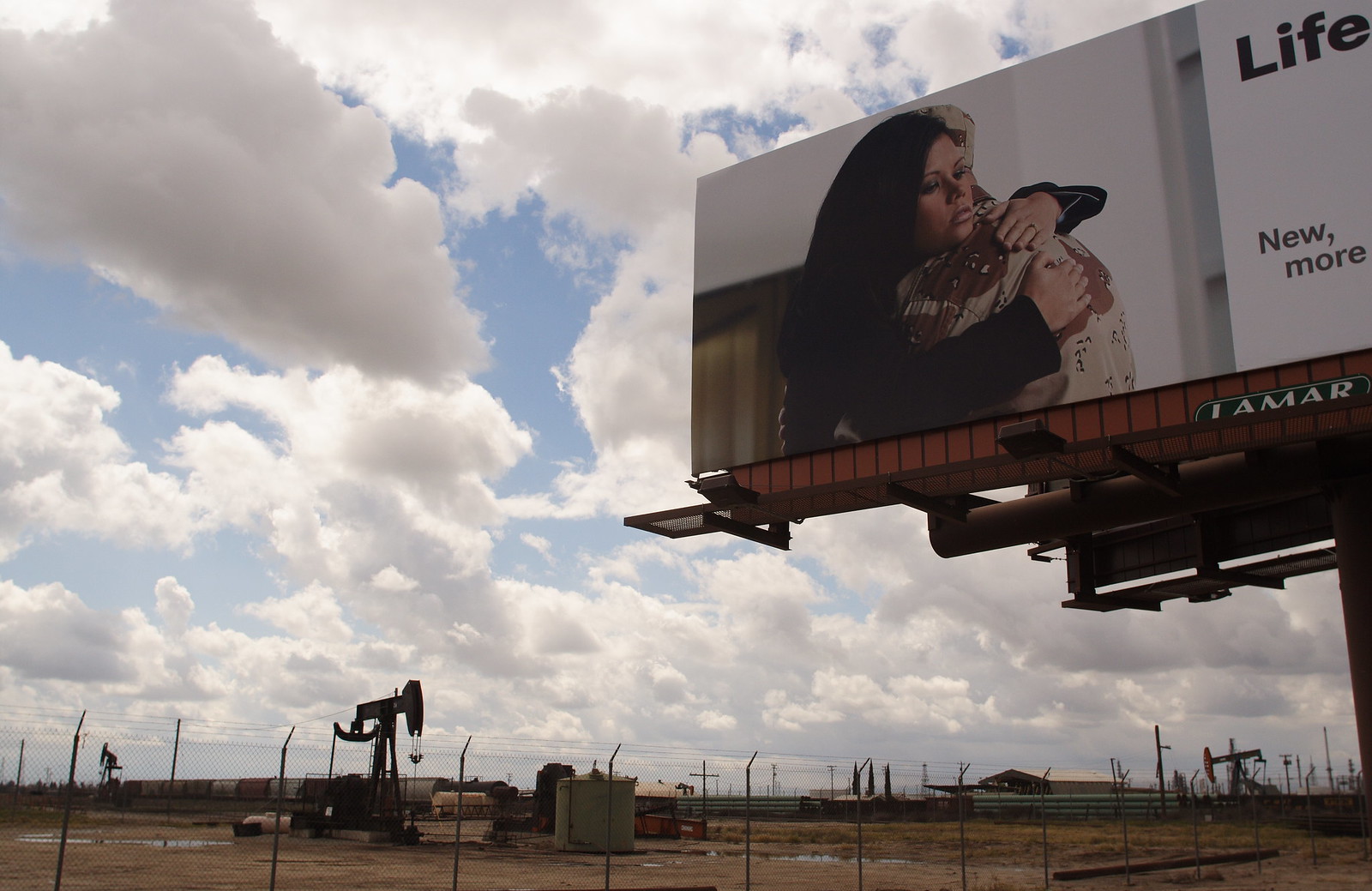The image captures a fragmented view of a billboard, with only its left edge visible as it protrudes from the upper right corner of the frame. Below the billboard, a fenced-in construction site dominates the scene, featuring a crane situated in the lower left section and a scattered pile of wood in the lower right. The majority of the composition is filled with an expansive sky, giving the impression that the photo is taken from a low vantage point looking upward. The peripheral elements, such as the construction site and the billboard, frame the sky, creating a juxtaposition between the industrial activities below and the open space above.